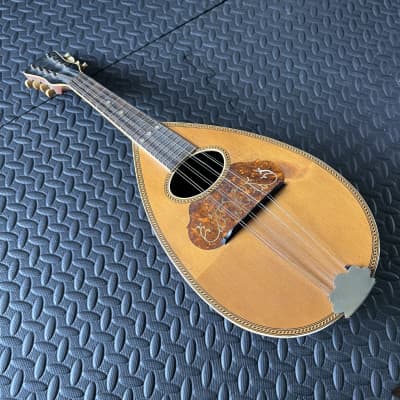This photograph captures a stringed musical instrument identified as a mandolin, characterized by its teardrop-shaped, long, oval base and a smaller body compared to a typical guitar. The instrument, which has eight strings, is situated diagonally across the frame, extending from the top-left corner to the bottom-right corner. Its composition includes a light beige wooden color with a darker shade around the sound hole, and a decorative border. The mandolin rests on a metallic, possibly tiled surface that features an intricate pattern, adding an additional layer of detail to the image.